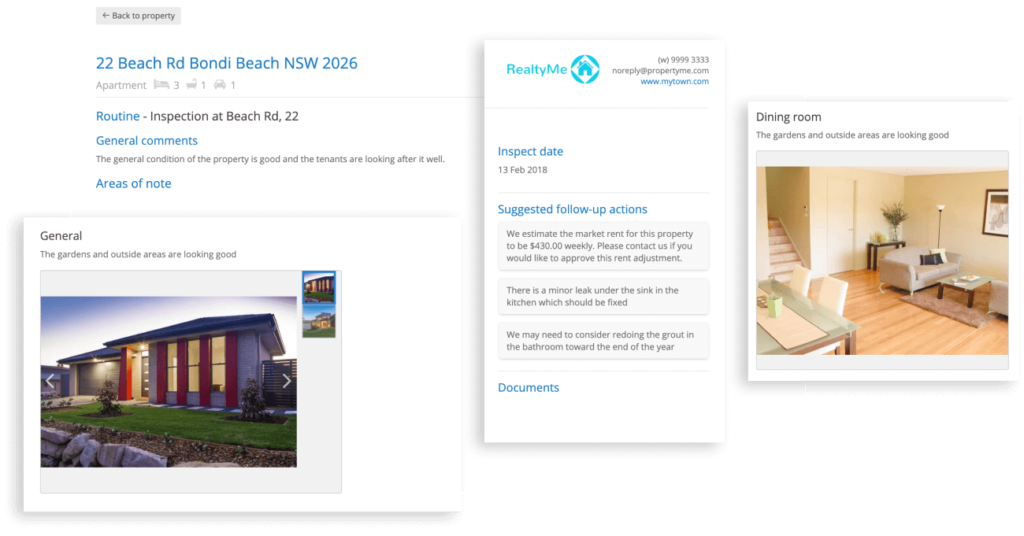A detailed screenshot capturing a property inspection report for 22 Beach Road, Bondi Beach, New South Wales, 2026. At the top, there is a light gray banner with a back arrow icon labeled "Back to Property."

Below, in bold blue text, "22 Beach Road, Bondi Beach, New South Wales, NSW 2026," is displayed, accompanied by categorizations: "Apartment, Routine, General Comments, Notes of Area." Adjacent to "Routine," in dark gray text, it reads "Inspection at Beach Road 22."

Further down, a white-background section labeled "General" in gray text remarks, "The gardens and asset areas are looking good." This area features photographs depicting various angles of the house, including the lawn and the sky, as well as two smaller stacked images showcasing the property from different perspectives.

A vertically aligned rectangle labeled "Realty Me" details an inspection conducted on February 13, 2028, with sections for "Suggested Follow-Up Actions" and "Documents," all highlighted in blue text.

Lastly, another square section titled "Dining Room" comments, "The gardens and asset area are looking good," and displays an interior view of a living and dining space with a small stairway leading upwards.